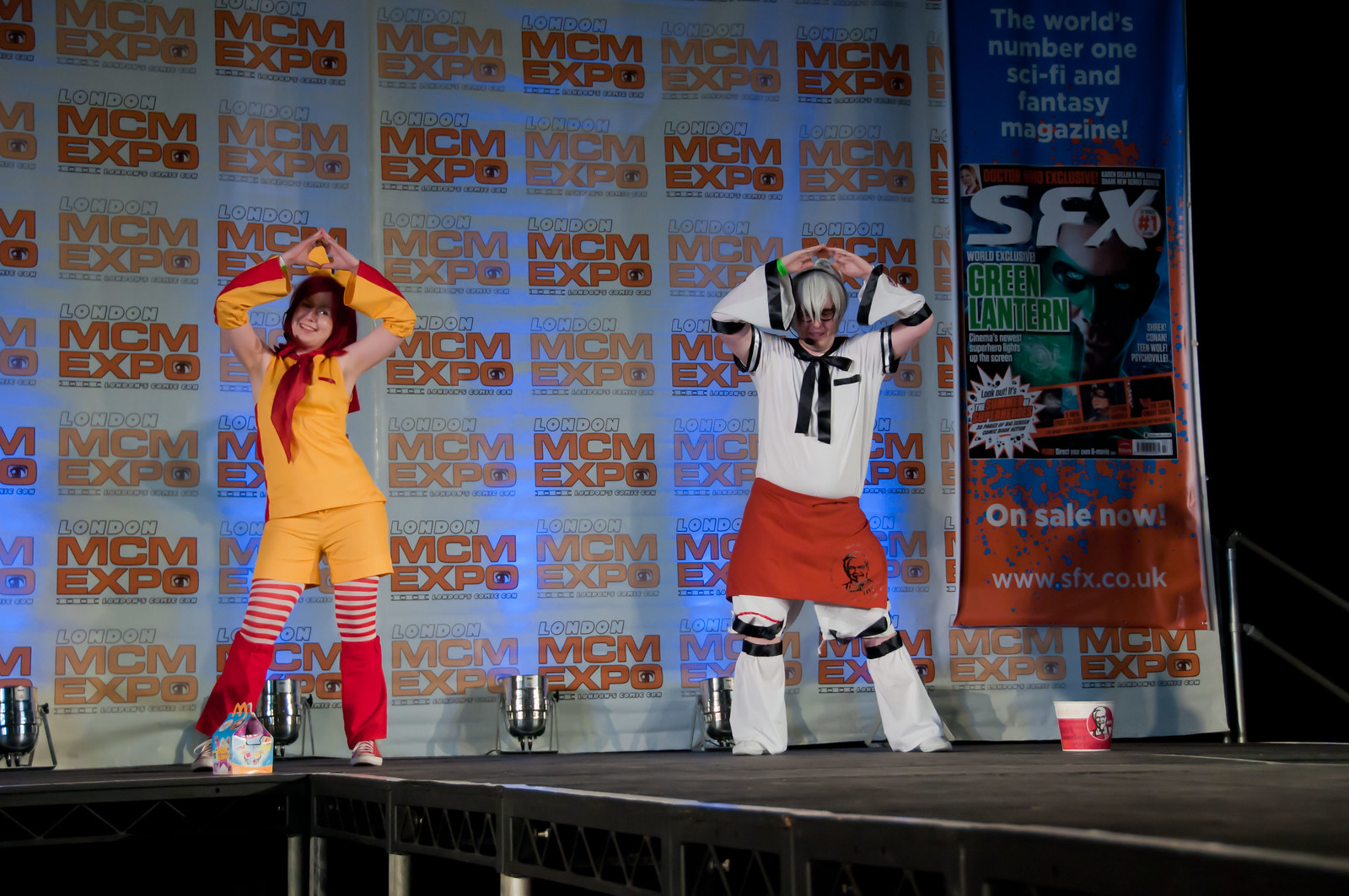In this rectangular image, two people, cosplaying on stage at the London MCM Expo, capture the spotlight with their lively performance. The stage at the bottom of the image features a runway extending diagonally from the bottom right corner upward to the left. The left performer, a woman with bright red hair, is adorned in a McDonald's-themed outfit featuring a yellowish-orange shorts and top combo, a red bandana around her neck, red and white striped tights, and yellow and red cutoff sleeves on her arms. In front of her is a Happy Meal as she dances energetically. To her right, a man dressed as Colonel Sanders from KFC is highlighted by his white and navy blue shirt and pants, accompanied by a navy blue ribbon bow and a red skirt with a logo. His short silver hair complements his white and blue cutoff sleeves. In front of him sits a bucket of KFC. Both individuals have their hands raised above their heads, fingers forming a triangle, as they sway their hips, seemingly lost in the rhythm of the dance. The backdrop includes banners for the London MCM Expo and a large sign promoting "SFX," the world's number one sci-fi and fantasy magazine, featuring their website www.sfx.co.uk and magazine imagery.